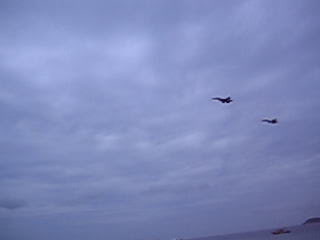This landscape-format, color image captures a pair of military jets flying low beneath an overcast sky. The image, likely taken with a phone, is poorly executed and low resolution. Both jets are positioned diagonally across the frame, with one slightly in front of the other. The sky is dense with solid, white cloud cover, featuring slight ripples. In the bottom right corner, the horizon introduces a coastal scene with water and a boat, hinting at the photo's angled perspective. The dark, featureless jets are viewed from below and the side, making them difficult to identify by branch of service, though the wing shapes and pointed noses are discernible. The aircraft are heading left, maintaining a rhythmic formation against the muted backdrop.